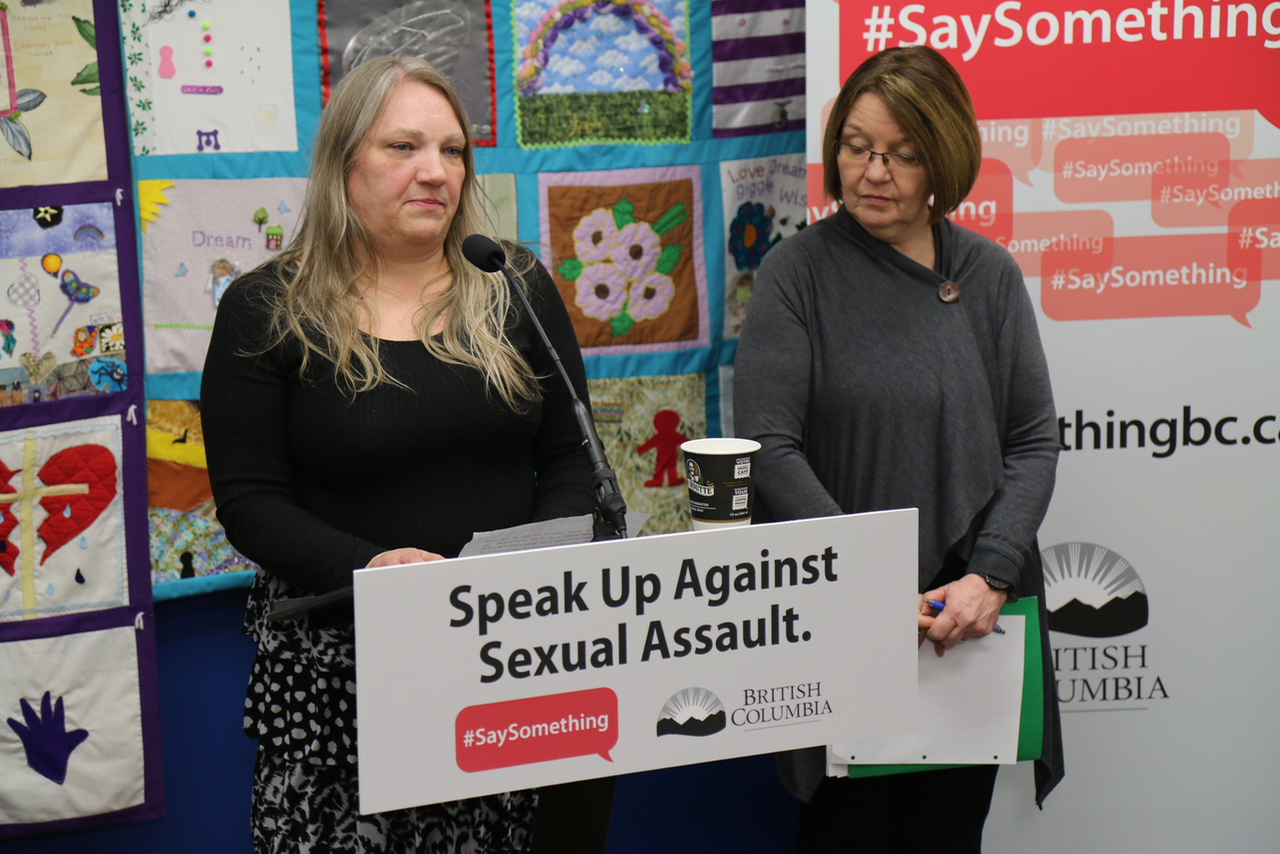The image captures a scene from a sexual assault awareness seminar. At the forefront, a podium prominently displays a sign reading "Speak Up Against Sexual Assault," with a red speech bubble beneath it containing the white text "#SaySomething." To the right of this, the podium features the British Columbia logo depicting mountains and a sunrise, with the text “British Columbia” next to it. At the podium stands an older woman in her 50s or 60s with long dirty blonde hair, dressed in a black sweater and a black-and-white dress. She is holding notes and speaks into a microphone extended from the podium. Beside her is another woman with short brunette hair, glasses, and a gray sweater, holding papers and pens with her hands folded. In the background, a white wall displays multiple transparent red speech bubbles, each bearing the hashtag "#SaySomething." Additionally, there are sections of a quilt with varied patterns, including flowers and a rainbow, adding a touch of color and texture to the setting. A steaming coffee cup rests on the podium, underscoring the seminar's informal yet earnest atmosphere.